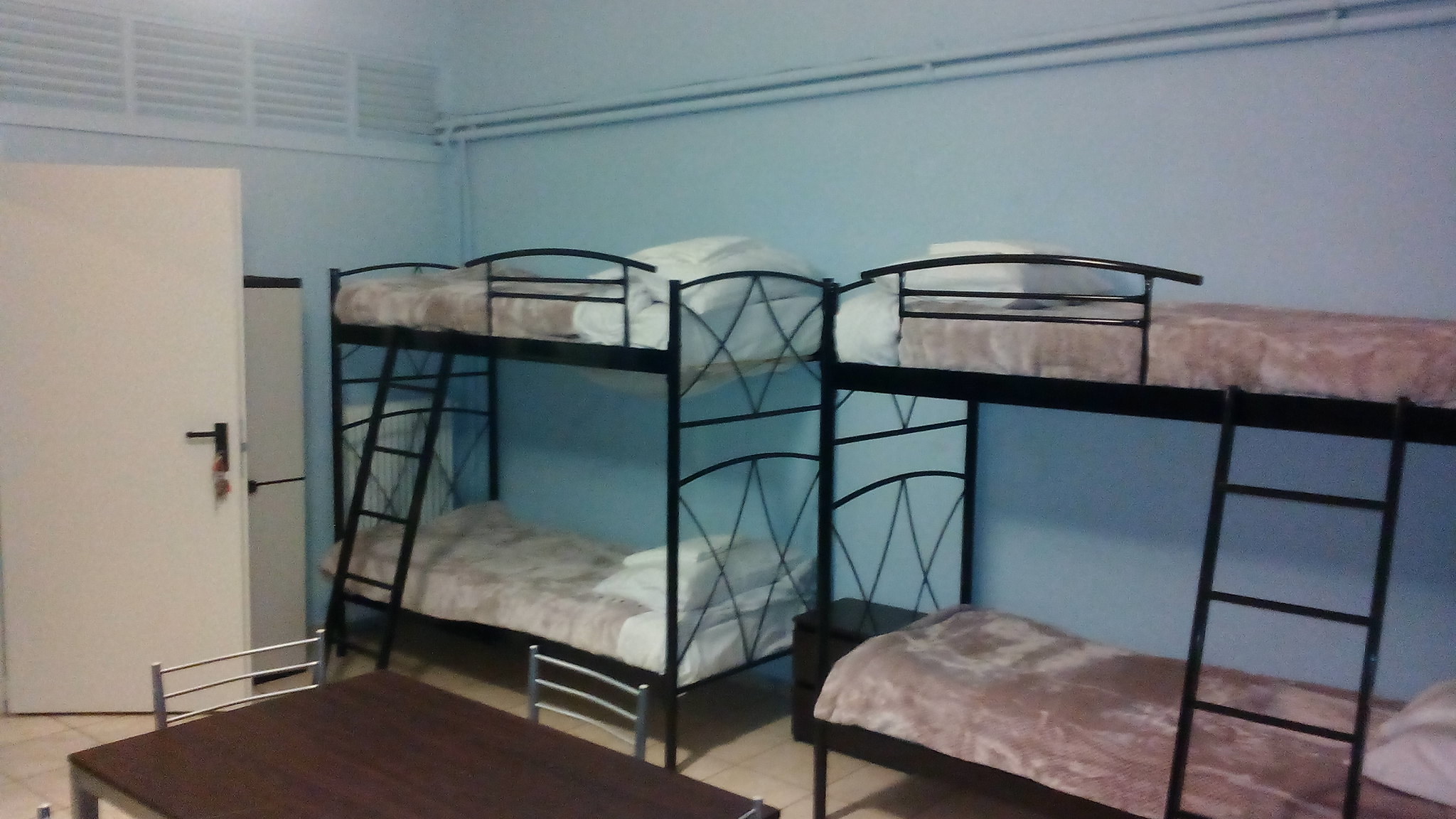This image depicts the interior of a spacious room, potentially a dormitory, hostel, or bunkhouse, with walls and ceiling painted in a soothing blue hue. Central to the scene are two sets of black metal bunk beds, each featuring sturdy, wrought iron frames and ladders attached at either end. Each bed is neatly dressed in grayish-brown, crushed velvet-like blankets, complemented by white pillowcases and sheets. 

In front of the bunk beds, against the blue wall, there stands a wooden table equipped with metal legs surrounded by two silver metal chairs. A large, white door with a black pull-down handle is visible on the left side of the room, just adjacent to a painted-over ventilation strip. The overall orderly arrangement and consistent furnishing suggest a well-maintained, communal sleeping space.